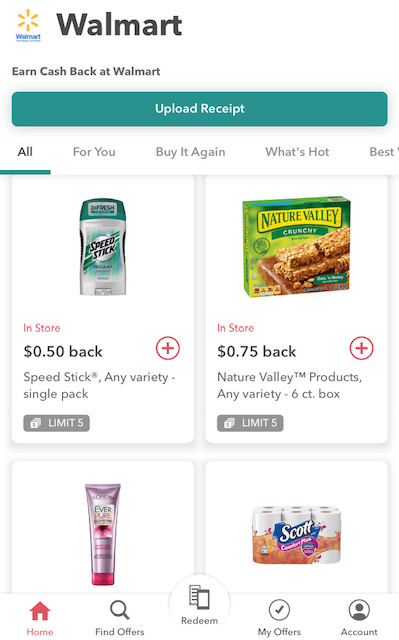At the top of the image, there is a banner featuring the Walmart logo on the top-left side, accompanied by the text "Earn cash back at Walmart." Below this banner, there is a large, dark blue button that says "Upload receipt."

The main section of the image has a white background and features several categories: “All For You,” “Buy It Again,” “What’s Hot,” and “Best,” each of which is underlined.

On the left side of the image, there is an image of a stick of deodorant with a bluish-green cap and logo on the front. Below this product, the text indicates "In-store 0.50 back." There is a red circle with a plus sign in the middle, and the text reads "Speed Stick, any variety, single pack, limit five."

On the right side, there is a green box with the text "In-store 0.75 back" followed by another red circle with a plus sign and the description "Nation Valley product, any variety, six-count box, limit five."